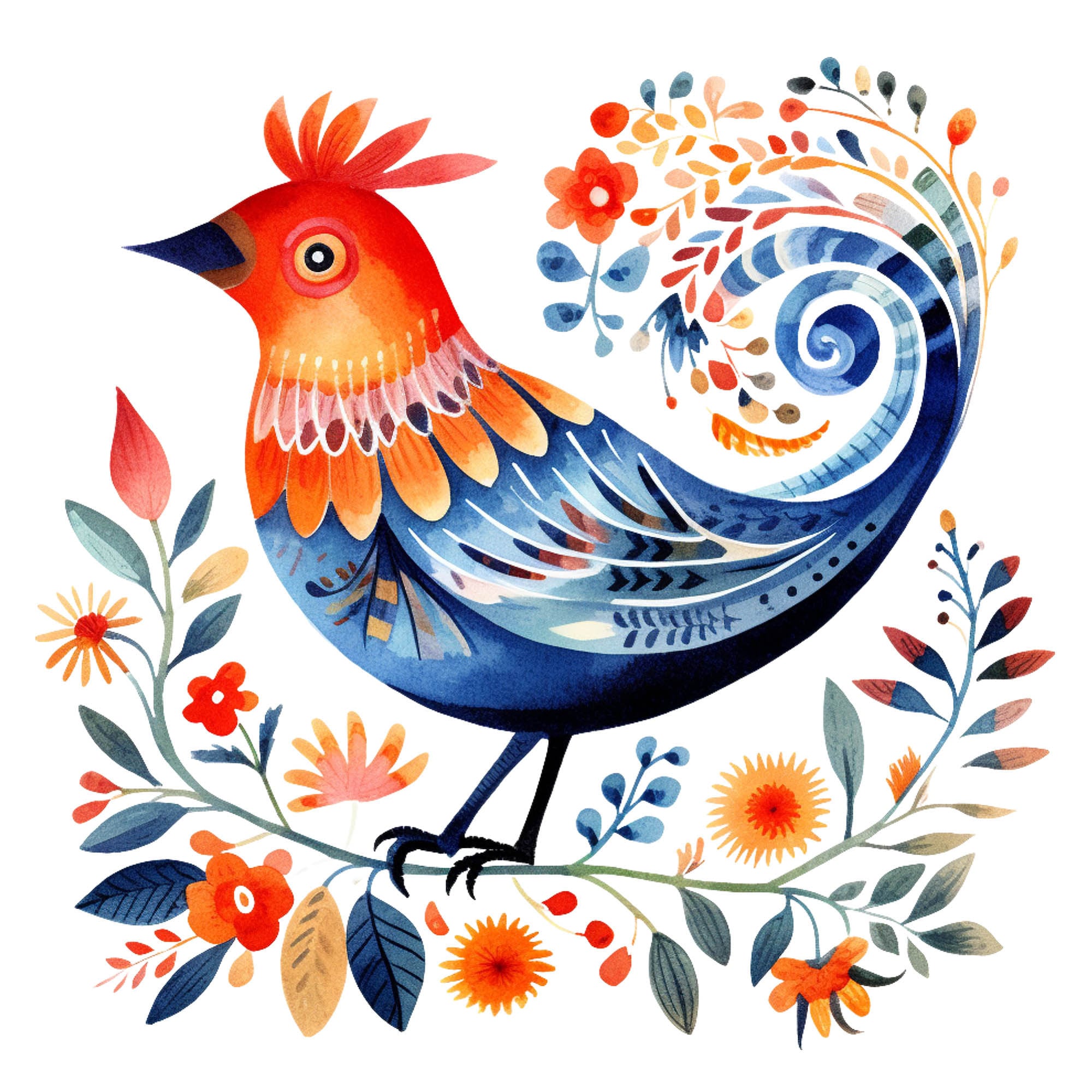This image showcases a detailed and vibrant piece of folk art painting that evokes the style of German Pennsylvania Dutch. The artwork features an ornately colored bird, predominantly orange and blue, with a pinkish-purple ring around its neck and a dark beak. The bird's head is adorned with five orange feathers, and its eye is notable for being a small black dot. The bird's wings are decorated with intricate patterns of dots and small leaf-like designs. A striking feature is its tail, which elegantly curls around and transitions into a cascade of flowers in shades of orange, yellow, brown, and blue.

The bird is perched gracefully on a flowering branch, which arcs upward on both sides of the bird. This branch is a blue-green hue and is covered in an assortment of colorful flowers and leaves, including shades of orange, blue, peach, teal, dark red, and dark blue.

The background of this folk art piece is a simple, clean white, which allows the vivid colors of the bird and the branch to stand out strikingly. The bird's body is a mix of bluish-black plumage, and its face features vibrant orange-red tones. The bird's eye is distinctive, with a dark black center surrounded by white and encircled by rings of orange and red. This intricate and lively painting captures the essence of traditional folk art with its rich palette and detailed motifs.